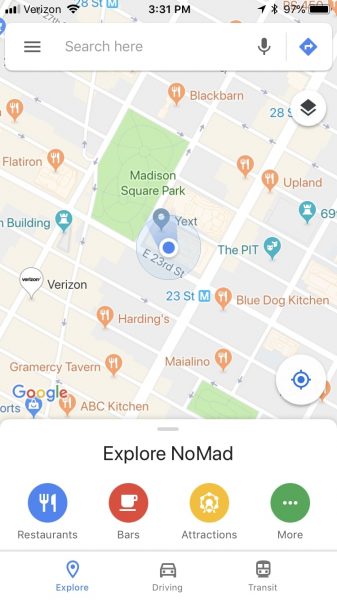This is a screenshot captured on someone's phone, showcasing a map of the Chelsea area in Manhattan, particularly the Nomad neighborhood, an abbreviation for North of Madison Avenue, coined by real estate agents in recent years. The map highlights a variety of dining options, with several restaurants like Blue Dog Kitchen, Black Barn, and Upland prominently marked. A blue dot on the map indicates the user's precise location, suggesting they might be searching for a nearby restaurant to visit.